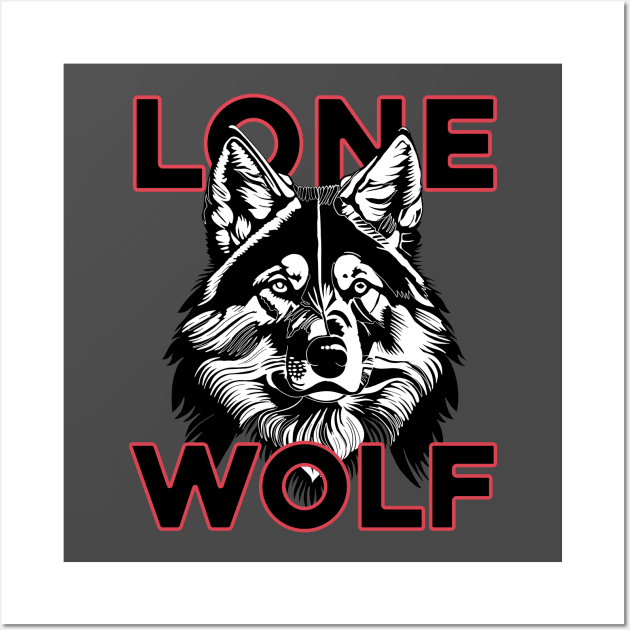The image showcases a striking graphic poster featuring a highly detailed black and white wolf's head, set against a dark gray background. Above the wolf's head, the word "LONE" is prominently displayed in bold, capitalized text with a neon-like pink or red outline, partially intersected by the wolf's ears. Below the wolf's head, the word "WOLF" is similarly styled with a bold black typeface outlined in pink or red, creating a glowing effect. The wolf's head is intricately drawn, capturing the texture of its fur and its facial features, giving it a piercing yet not menacing look, almost friendly. The overall design is modern and edgy, with the contrasting colors and bold fonts making the phrase "LONE WOLF" stand out vividly.